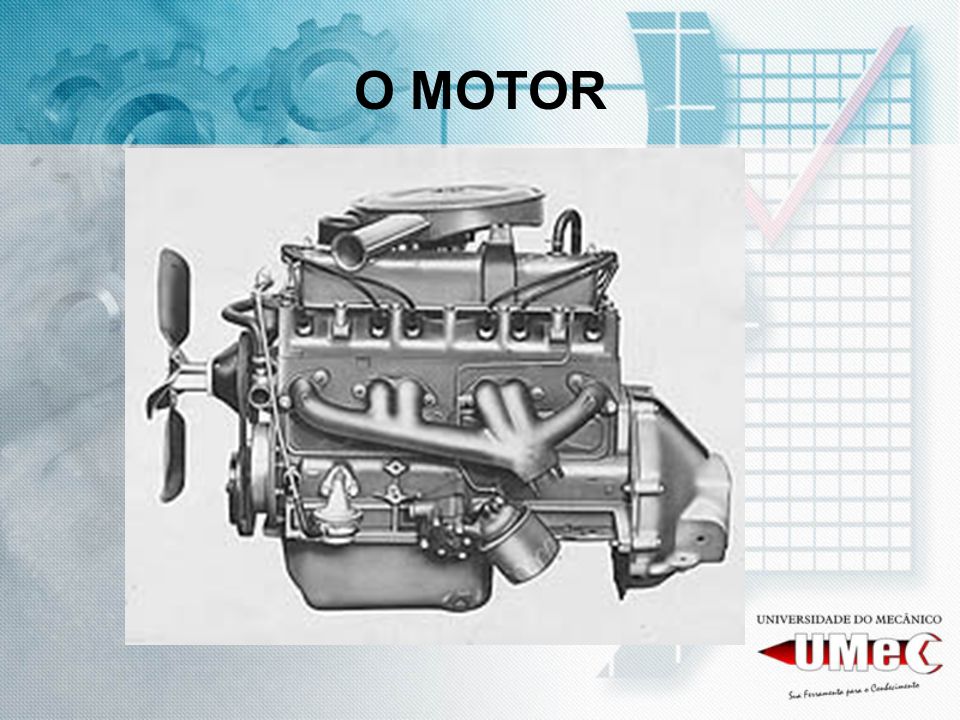This image features a detailed depiction of a silver car motor set against a predominantly white background with light blue and gray elements. The top fifth of the image displays a light blue and white horizontal section, featuring the text "O motor" in bold, black capital letters. Superimposed on this section are illustrations of two blue gears or flywheels. Beneath this, a large, detailed motor dominates the center, showcasing various components such as a fan on the left side, six wires likely leading to spark plugs, and an air filter pointing to the far left. The motor also includes visible gears, pistons, pipes, and what appears to be an oil tank underneath. On the right-hand side, the image includes a vertical strip resembling graph paper with a subtle check mark. In the lower right corner, the text "Universidad del Mecanico" and the acronym "UMEC" appear in a combination of white and black letters, with some additional small, indistinct text underneath, possibly in Spanish.